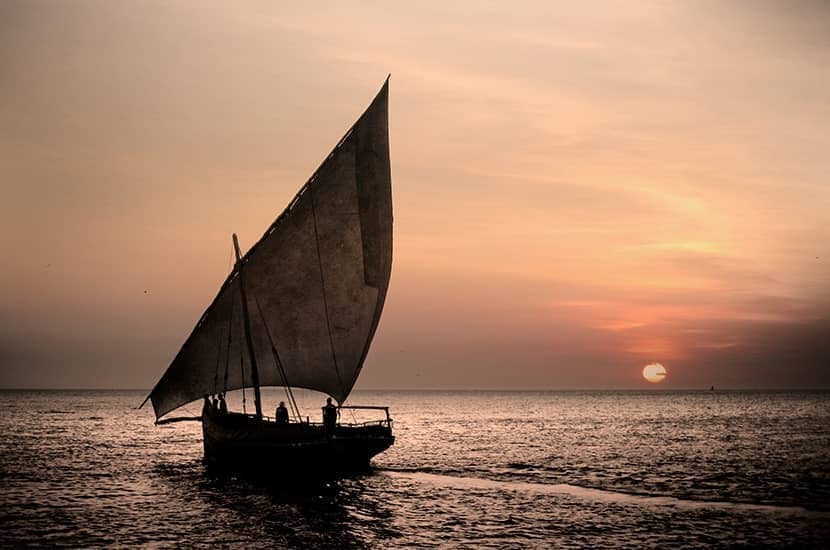In this somewhat older, slightly compressed photograph taken outdoors, we witness a serene seaside sunset. Dominating the scene is a calm sea that stretches out into the hazy horizon. To the right, a softly glowing orange sun nears the horizon, casting a beautiful orange hue across the surrounding clouds. On the left, a sailboat cuts through the water, leaving a small wake behind. The sailboat, shrouded in darkness with only its white sail visible, is silhouetted against the dimming light, which makes details sparse but outlines the presence of two standing figures onboard. Far in the distance near the setting sun, a small triangular-shaped sailboat can just be made out on the horizon, adding depth to the vast scene. Above the left sailboat, a lone black dot—possibly a bird—can be seen against an otherwise clear sky. The overall color palette includes shades of orange, yellow, pink, gray, and black, tying together this tranquil seascape at sunset.